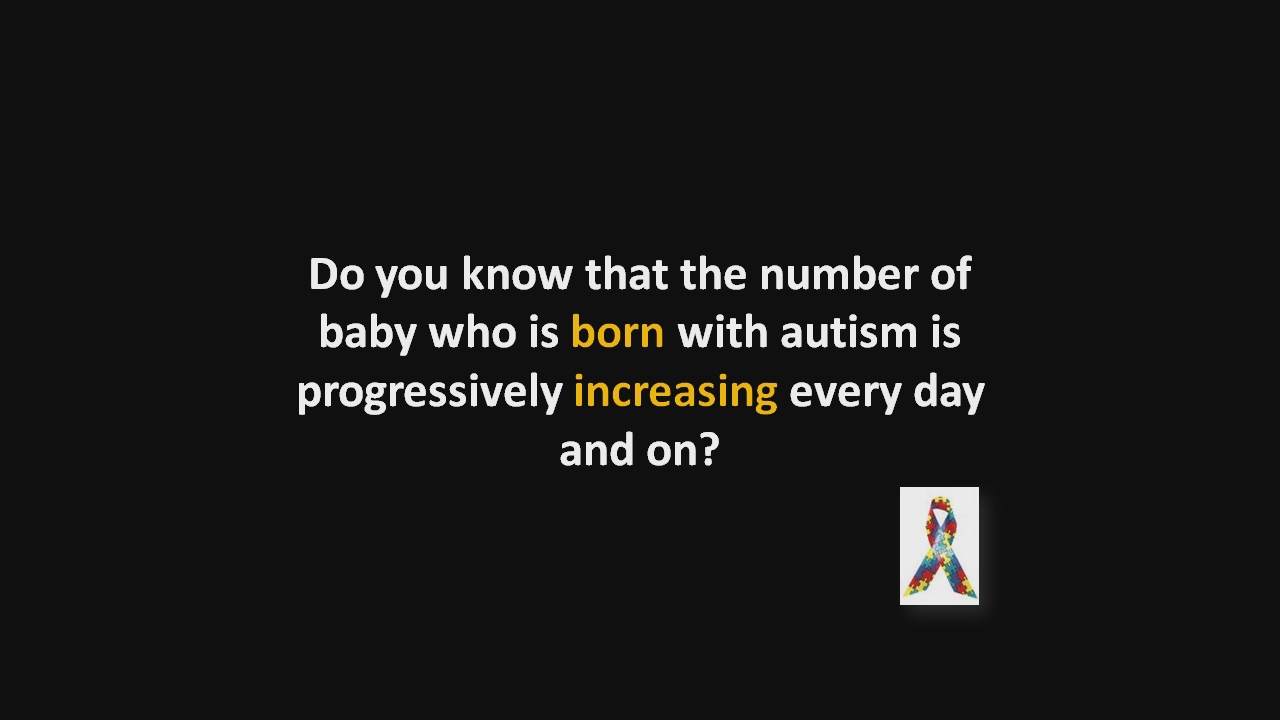This image features a public service announcement on a completely black rectangular background. The central text, displayed in white font with the words "born" and "increasing" highlighted in yellow, reads: "Do you know that the number of babies born with autism is progressively increasing every day and on?" The text is arranged across four lines, with the final line simply containing the words "and on." Below the text, positioned centrally, is a multicolored ribbon symbolizing autism awareness. This ribbon, comprised of blue, red, yellow, and light blue puzzle pieces, sits within a small white rectangle spaced slightly below the word "day" and before "and on."